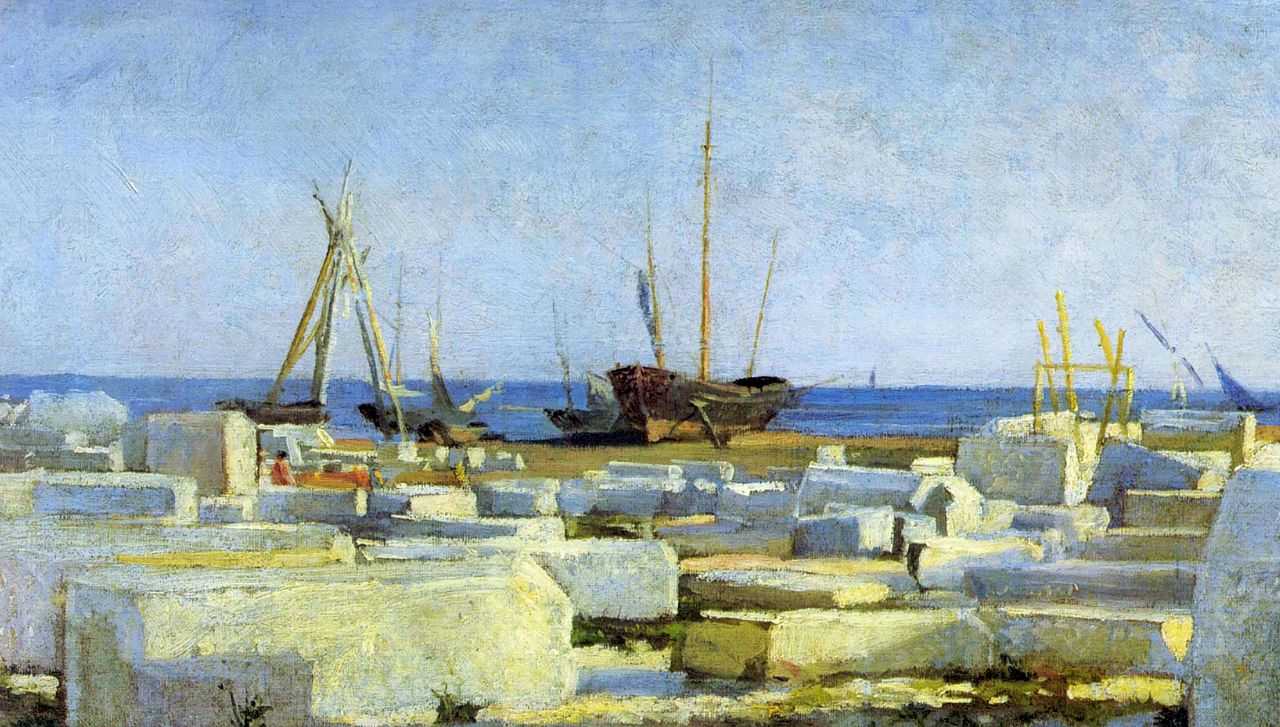This painting captures an outdoor maritime scene by the ocean during daylight. Centered prominently is a large, historical sailing ship, distinguishable by its three towering masts that remain bare, with no sails unfurled. The ship's hull is predominantly black with complementary tan accents near the bottom. The ship rests in a dry dock on land, surrounded by numerous white rectangular stone blocks, some piled high and one featuring a set of steps.

In the left foreground, a teepee-like wooden structure, possibly for boat repairs, stands out. Various other older ships, all with their sails down, are docked nearby, suggesting a bustling shoreline. The right end of the painting subtly includes a windmill, adding to the historical ambiance.

The background showcases a serene blue sky adorned with scattered clouds, blending seamlessly into the expansive ocean horizon, which stretches across the entire width of the canvas. The ocean and sky dominate with hues of blue, contrasting with the earthy tones of the stones, sand, and ships, while sporadic patches of green grass add a touch of verdant color to the composition.